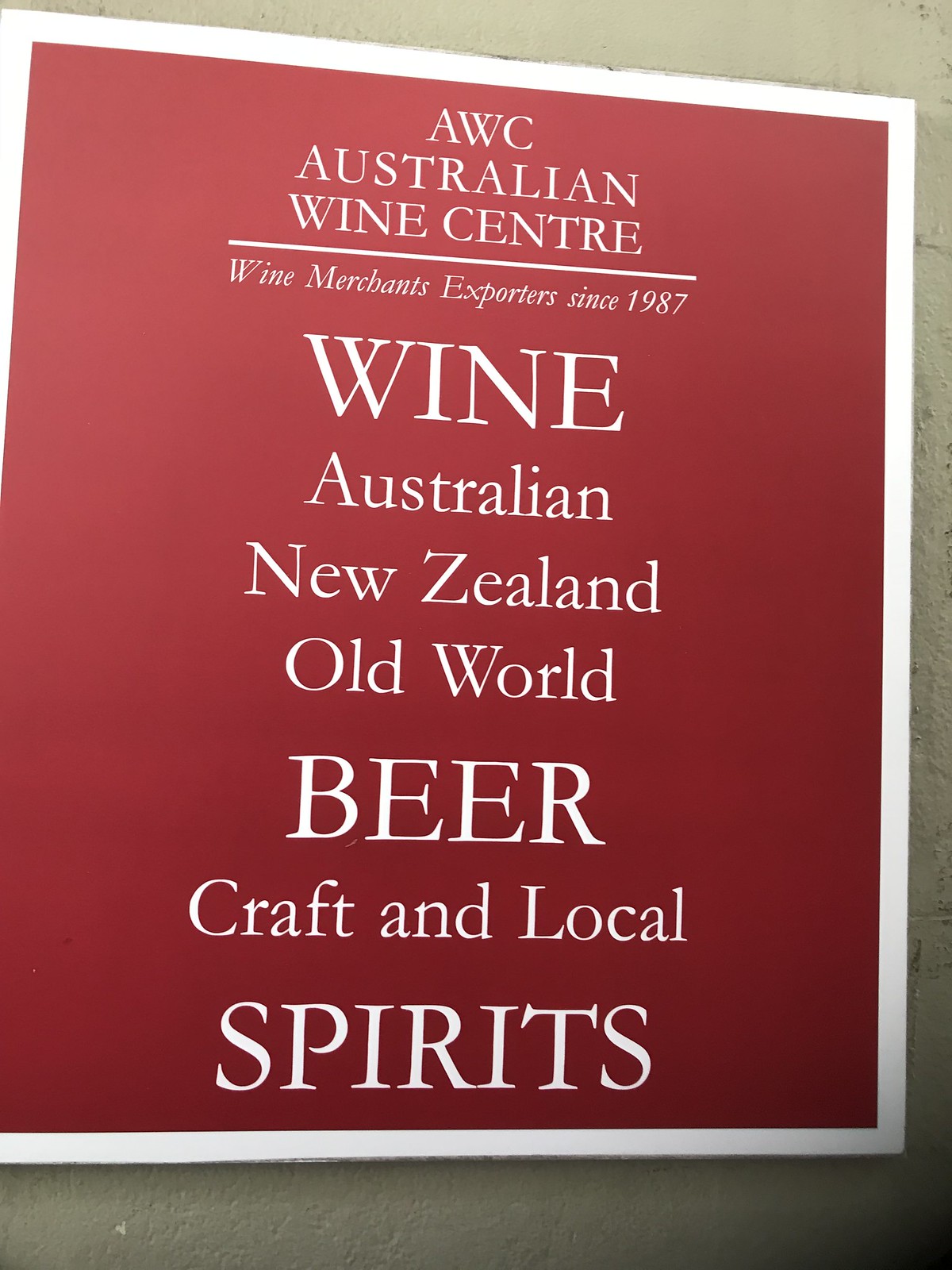The image features a prominently detailed, red and white sign mounted on a dingy white wall. The sign has a white border and white capitalized letters set against the red background. At the very top, it reads "AWC" followed by "Australian Wine Center." Beneath this, separated by a white line, it states "Wine Merchants Exporters Since 1987" in smaller text. Further down, larger text lists "Wine," and below it in smaller letters: "Australian," "New Zealand," and "Old World." The progression continues with "Beer" written in larger letters, and then "Craft and Local." At the very bottom, the sign proclaims "Spirits" in large bold letters. The overall arrangement of the text gives a clear emphasis on different types of beverages offered, with key terms like "Wine," "Beer," and "Spirits" standing out prominently.